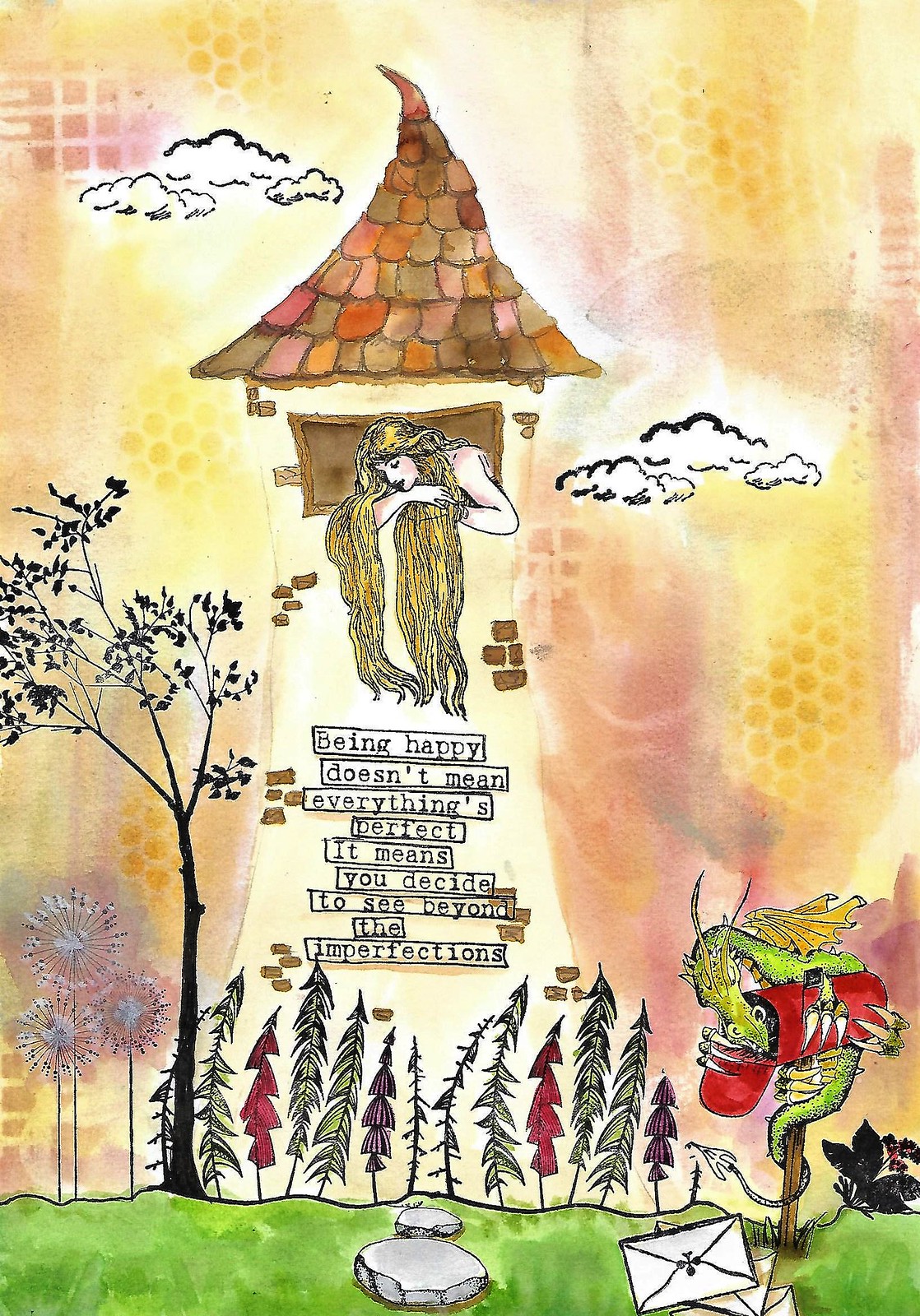This vibrant and whimsical painting features a picturesque scene centered around Rapunzel's tower. The tower, made of bricks with a distinct pointed roof, stands tall amidst a surreal landscape. Rapunzel, with her long blonde hair cascading out of a window, is depicted in a fluid watercolor style that merges sketching and painting. Surrounding the tower are various colorful trees in hues of red, green, and purple, alongside a taller black tree to the left. In front of the tower, a mischievous green dragon entwines a wooden post topped with a red mailbox, taking a bite as letters spill onto the green grassy ground below, dotted with stepping stones. The sky is a stunning blend of yellow, pink, and purple, accentuated with white and black clouds, contributing to the dreamlike quality of the artwork. Notably, there are three oversized dandelions taller than some of the trees on the left side of the image. The painting also features an inspirational quote: "Being happy doesn't mean everything's perfect, it means you decide to see beyond the imperfections," written in the middle of the tower. The bright colors and imaginative details, like the sky peeking out behind the tower and the mix of abstract elements, bring a lively yet serene atmosphere to the scene.